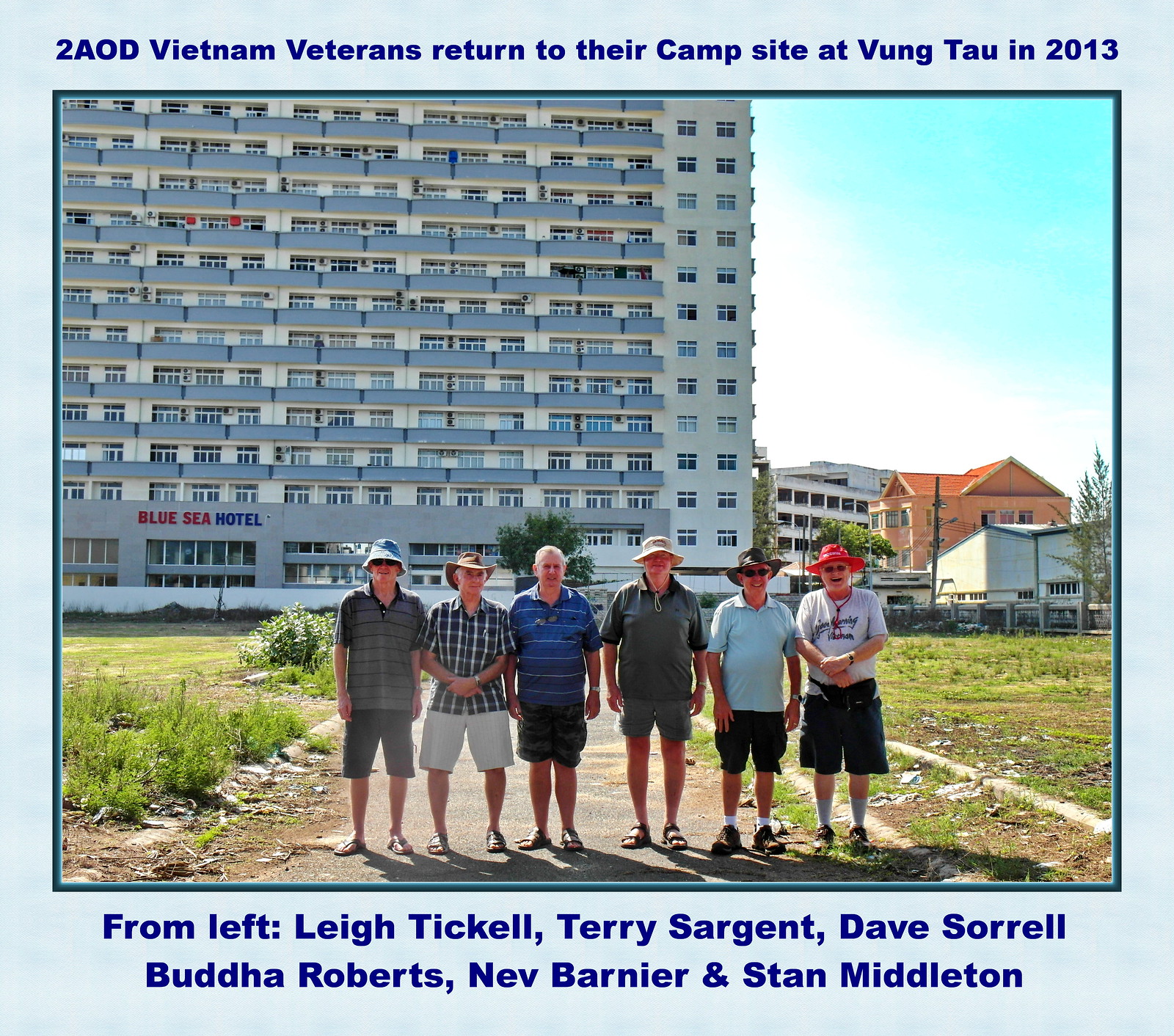The photograph depicts six older men, likely in their 60s or 70s, all dressed in shorts and short-sleeve shirts, standing outside in front of a large building identified as the "Blue Sea Hotel." The men, who appear to be Vietnam War veterans, are positioned left to right as follows: Lee Tickle (gray shirt with black stripes), Terry Sargent (white and black striped shirt), Dave Sorrell (blue shirt with white stripes), Buddha Roberts (gray shirt), Nev Barnier (light blue shirt), and Stan Middleton (white shirt with writing). Five of the men are wearing hats, while Dave Sorrell, the third man, is not. The background includes a blue sky with clouds, additional buildings, and some grass and shrubs on the ground. The top of the image reads, "Two AOD Vietnam veterans returned to their campsite at Vung Tau in 2013," and the bottom lists their names. The image is framed by a light blue border.